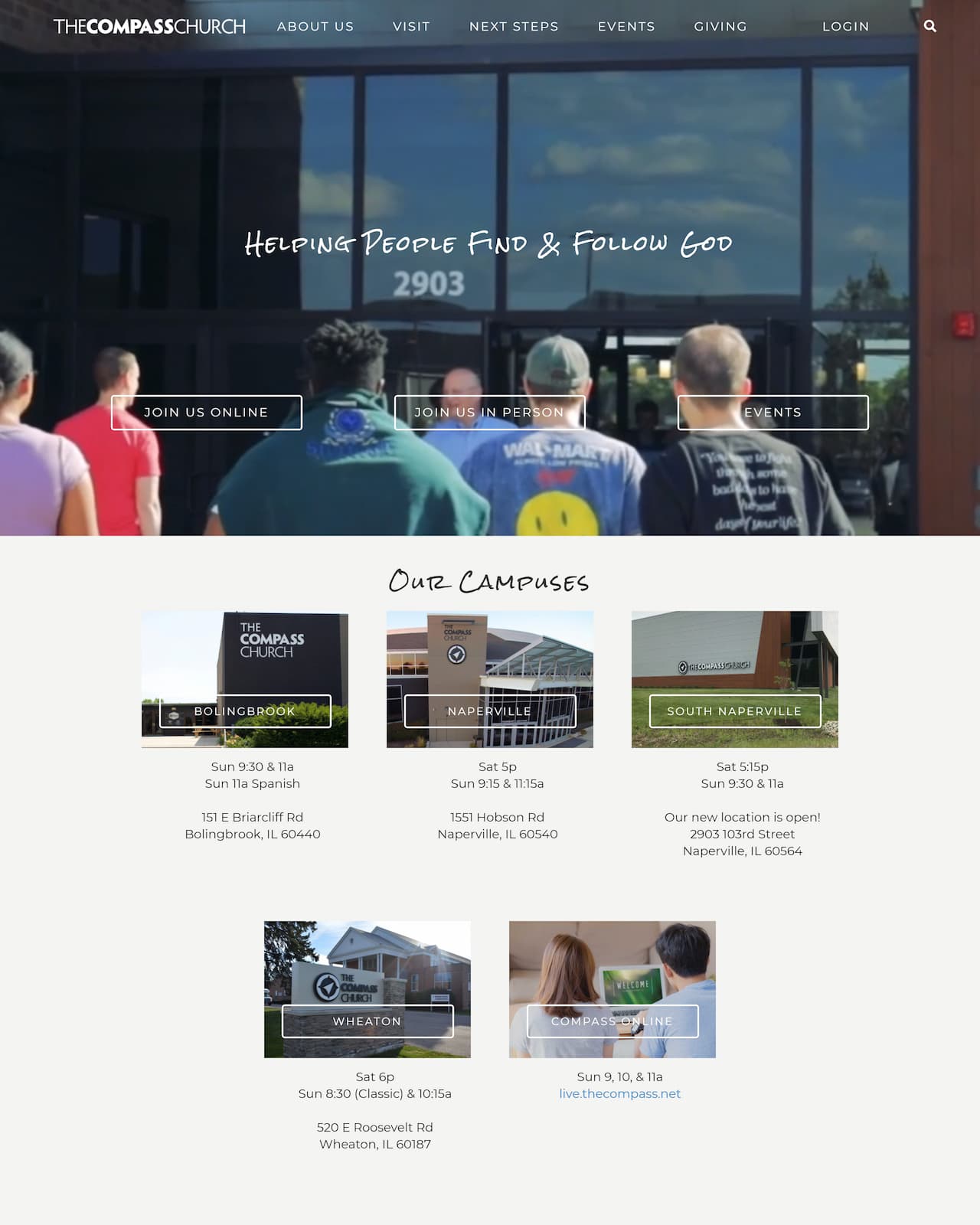The screenshot captures a comprehensive view of a webpage from The Compass Church. The top half of the screenshot features a photograph showing five men attentively listening to another man, presumably delivering a speech or presentation. Above this image is a menu bar with options: About Us, Visit, Next Steps, Events, Giving, and Login, accompanied by a magnifying glass icon for search in the upper right corner. Centrally located on the image is the church's mission statement: "Helping People Find and Follow God," followed by three interactive buttons: "Join Us Online," "Join This Person," and "Events." 

The bottom half of the screenshot focuses on The Compass Church's campus locations. It showcases five tiles, each representing a different campus with a corresponding photograph. The campuses listed are Bounce Back Book, Naperville, South Naperville, Wheaton, and Compass Online. Each tile also provides details such as dates and addresses for these locations.